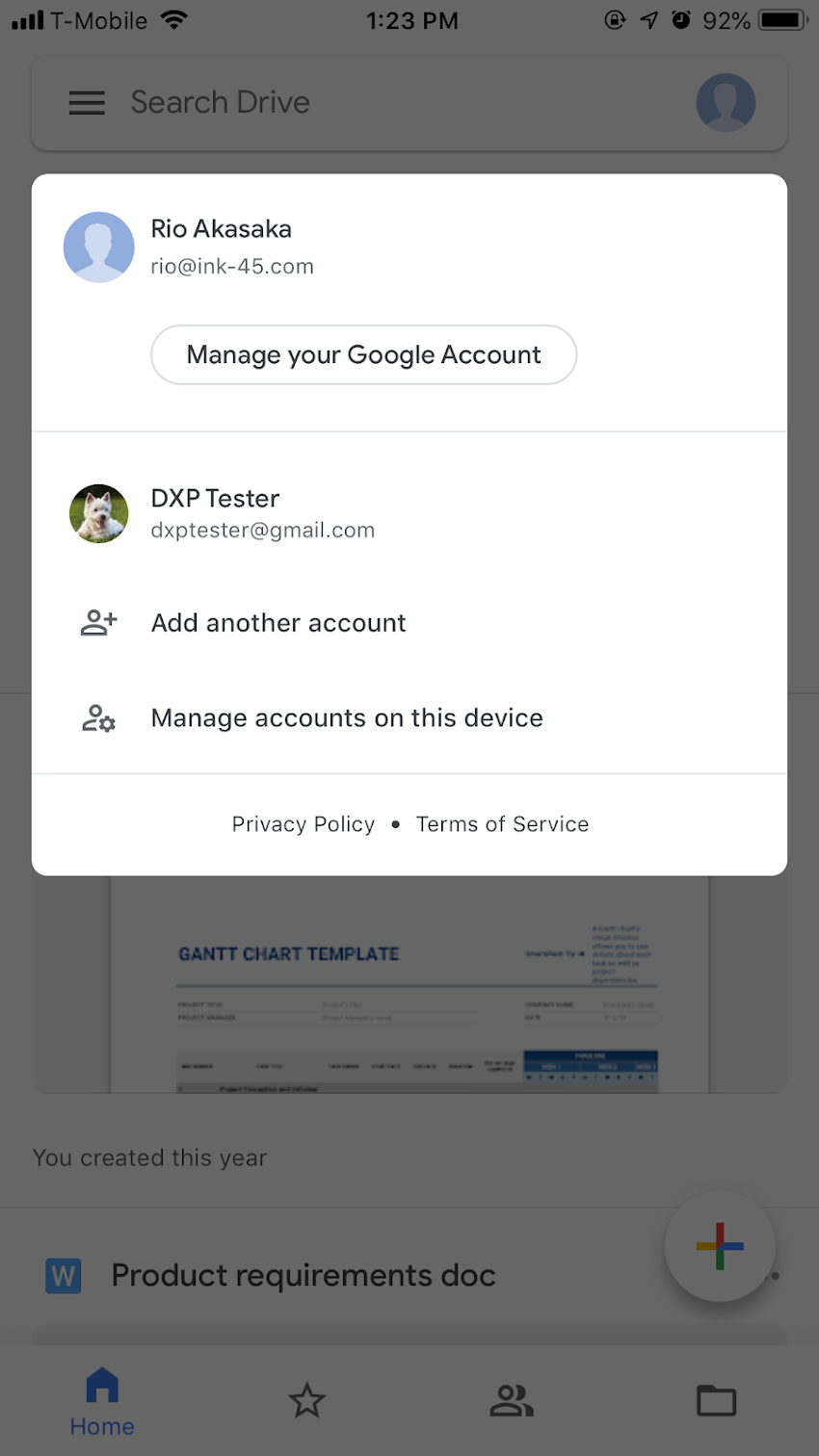This image captures a cellphone screen displaying a Google account management interface. The background of the screen is partially grayed out with an opaque overlay, making the underlying content faintly visible. Prominently, a white rectangular pop-up window is superimposed on the gray background. At the top of this window, "Rio Acasake" is displayed, followed by a URL link and the instruction to "Manage your Google account."

The pop-up window is divided into three main sections. The first section features a profile avatar of a small white dog, labeled "DXP tester," with the email address "dxp.tester@gmail.com" beneath it. The second section contains an icon of a human silhouette with a plus sign next to it, offering the "Add another account" option. The third section shows another human silhouette icon accompanied by a gear symbol, providing the "Manage accounts on this device" option.

At the bottom of the window, links to the "Privacy Policy" and "Terms of Service" are available. Extending below the pop-up, in the grayed-out area of the screen, a document titled "Product Requirement Doc" can be partially seen, along with a Google Plus icon located at the bottom right corner.